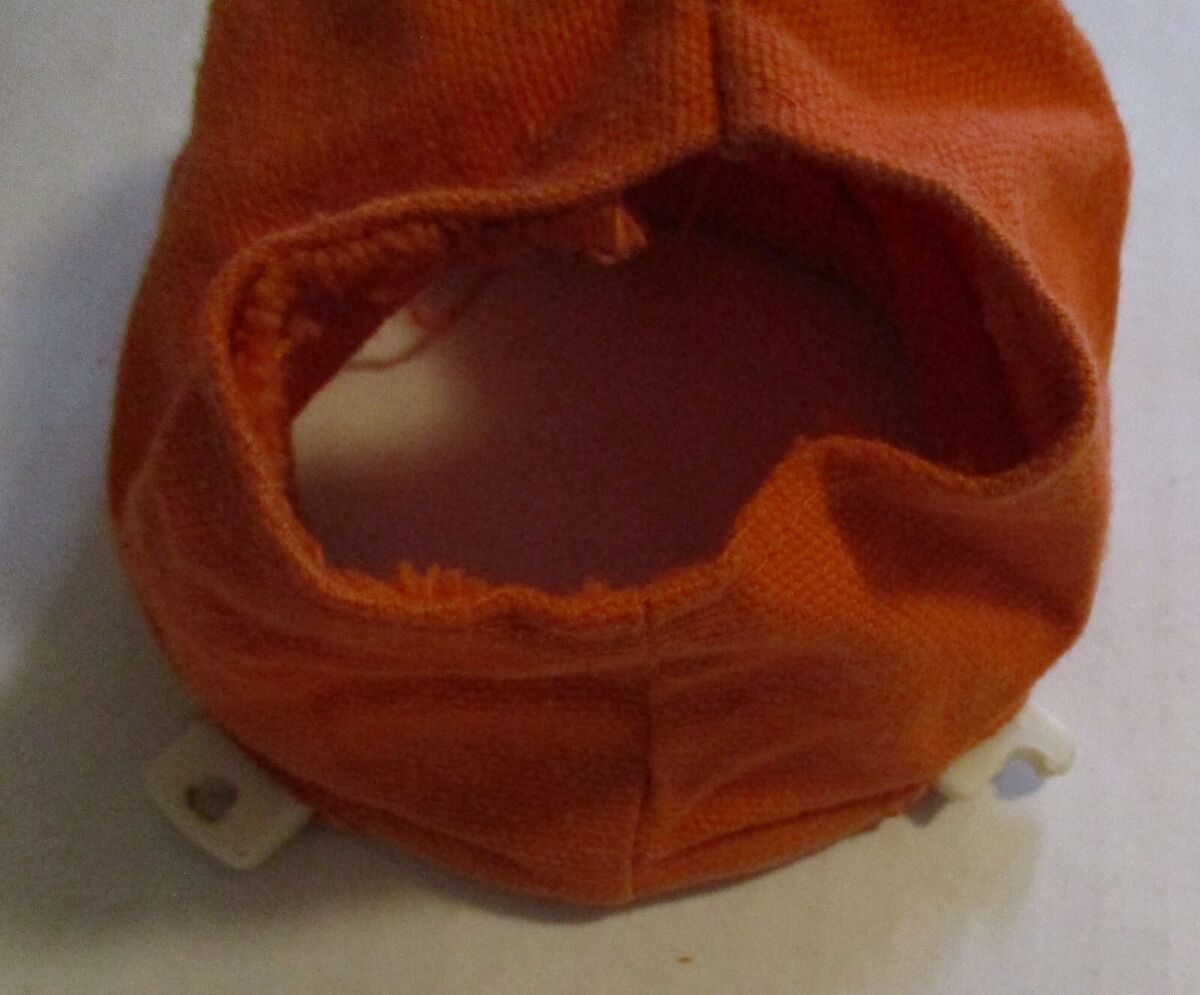This close-up photograph features a reddish-orange, knit fabric piece that resembles a homemade ski mask or a cut-off hood from a sweatshirt. The fabric is slightly translucent and worn, showing stray threads and signs of use. It has a circular opening in the center, bordered by sewn edges, allowing you to see through to a light gray or white background, possibly a countertop. The bottom edge of the fabric includes two rectangular white plastic tabs with holes in their centers; the left tab is intact, while the right tab appears broken. The entire piece is cut off at the top, giving it a somewhat rounded but incomplete shape.